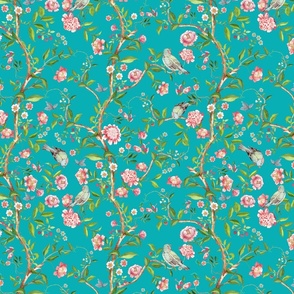This image showcases a delicate and intricate pattern that could be used for wallpaper or craft purposes. The design features a light teal blue background with a repeating motif of slender brown stems adorned with small green leaves. Interspersed among the foliage are dainty pink flowers, varying in size with some appearing as tiny polka dots. Additionally, the pattern includes small gray-brown and white birds scattered throughout the greenery. Some of the elements, such as a few leaves and flowers, appear to float unattached to the branches, enhancing the whimsical feel of the design. The pattern itself is meticulously repetitive, extending from top to bottom and left to right, ensuring a seamless and continuous visual effect suitable for various decorative applications.